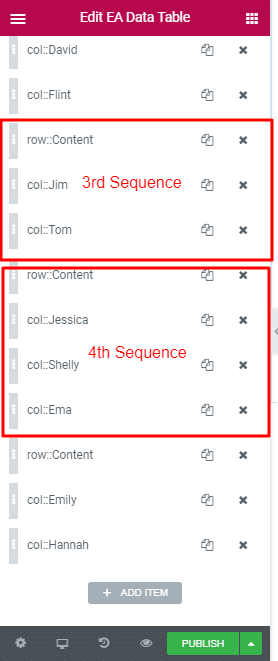The app interface displayed in the image features a maroon header titled "Edit EA Data Table." On the top left of the header is a menu icon, while the top right houses a grid view icon. The main section of the app, which boasts a white background, showcases a sequence of data entries. Each entry follows the format "Carl [Name]" or "Raw Content." The list includes:

1. Carl David
2. Carl Flint
3. Raw Content
4. Carl Jim
5. Carl Tom
6. Raw Content
7. Carl Jessica
8. Carl Shelly
9. Carl Emma
10. Raw Content
11. Carl Emily
12. Carl Hen

Towards the bottom of the screen, a grey button labeled "Add Item" is present. Additionally, there are two red-highlighted sections drawing attention to specific data entries. The first red square is labeled "Third Sequence" and highlights the entries: Raw Content, Carl Jim, and Carl Tom. The second red square, marked "Fourth Sequence," covers Raw Content, Carl Jessica, Carl Shelly, and Carl M.

The footer of the app includes several icons: Settings, Desktop View, Refresh, Hide, and a prominent green button labeled "Publish."